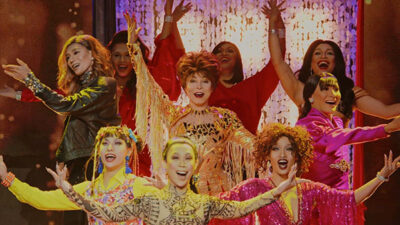The image captures a dynamic moment from what appears to be a musical or dance routine on stage, featuring a group of nine women energetically posing with outstretched and raised arms, exuding joy and excitement. The women, possibly in their 30s or 40s, are adorned in an array of vividly colorful and flashy costumes including hues of pink, red, gold, yellow, purple, lilac, and black. The scene is divided into three rows with three women each, creating a layered visual effect. The two women at the bottom left wear bright yellow outfits, while the one on the bottom right dazzles in a red sparkly robe. In the middle row, the leftmost woman sport a black leather jacket, the center woman captivates in an orange frilly ensemble, and the rightmost woman is dressed in vivid pink. In the back row, two women are seen in red attire, with one partially obscured by another performer. The background is a visually stimulating blend of pink with bright white lights, accompanied by brownish hues on either side, enhancing the stage-like setting. The central figure, a woman with short red hair, stands out as a potential lead, highlighted by her joyful expression and commanding presence. This image, devoid of any text, radiates a palpable sense of celebration and performance.